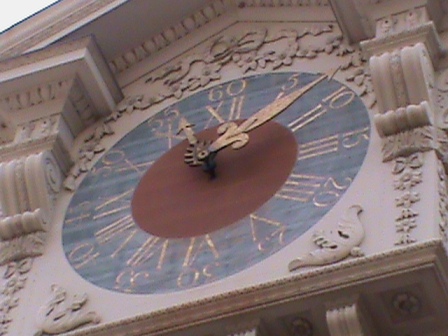The image depicts a large architectural clock mounted on a white, ornately decorated building. The clock face is light blue, adorned with golden Roman numerals and regular numbers marking every 5-minute interval up to 60, with gold hands. A distinct terracotta-red circle is present at the clock's center. The building features intricate floral and leaf designs and two pillar-like structures on either side, supporting a triangular pediment at the top. Above the clock, elegant carvings include a ribbon motif. The building's surface appears to be a pristine white-grayish hue, with the designs meticulously carved from rock. The time indicated on the clock is approximately 11:08.